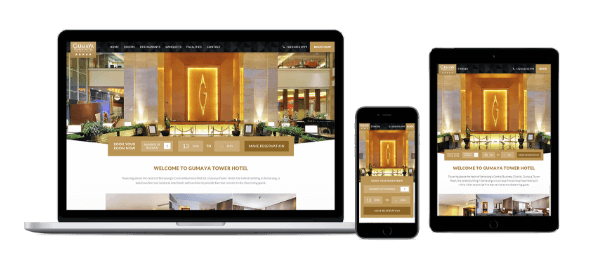The image showcases the responsive design of the Gumaya Tower Hotel's website across three different devices: a laptop, a smartphone, and a tablet. Each display presents the main page of the hotel's website, providing a clear view of the hotel's primary features and layout. On the laptop screen, the website is displayed in its fullest form, complete with a prominent high-resolution image of the hotel's main area, a date selection feature for booking visits, and a detailed summary paragraph about the hotel. The tablet display similarly includes these elements, effectively conveying the hotel's offerings on a medium-sized screen. However, the smartphone version, while still displaying the high-quality image and the date selection feature, omits the summary paragraph to accommodate the smaller screen size. This comprehensive side-by-side comparison highlights the website's consistency in delivering essential information across different devices while optimizing the layout for user experience on each platform.